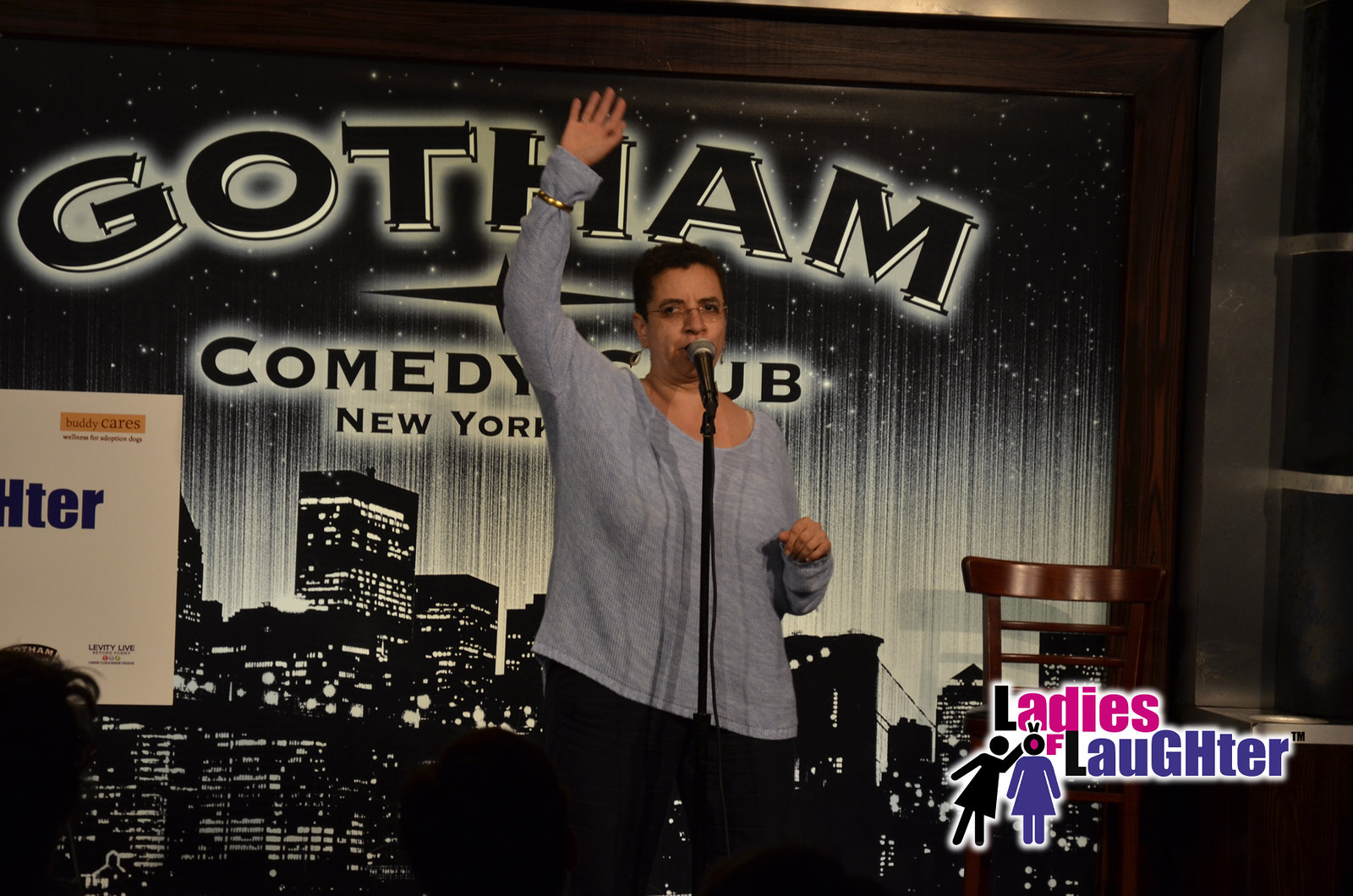This color photograph captures a woman performing stand-up comedy on stage at the Gotham Comedy Club in New York. She is dressed in a loose-fitting pale blue, long-sleeved shirt paired with black pants. A distinctive large gold bracelet adds flair, worn over the sleeve on her raised right arm. She has short black hair, or possibly pulled back, and wears small glasses. The backdrop features a striking black and white night-time city skyline, complete with towering buildings and the silhouette of the Brooklyn Bridge. A wooden chair is positioned to her left in the background. In the bottom right corner, a logo reads "Ladies of Laughter," with the 'L' in "Ladies" and "Laughter" in black, the remaining letters in "Ladies" in pink, and the rest of "Laughter" in navy blue. Beside the text are icons of a black stick figure woman and a blue woman silhouette, emphasizing the focus on female comedians.